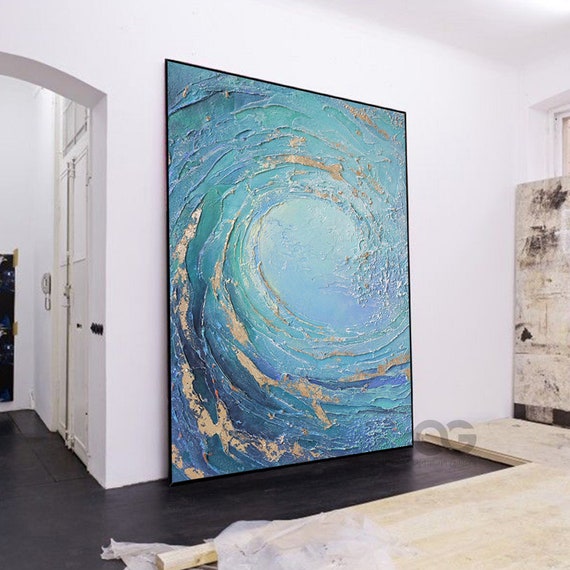The image depicts the interior of a house, centered around a prominent piece of abstract artwork. The room is spacious and well-lit with white walls and a dark brown hardwood floor. At the center, a large rectangular painting framed in black leans against a white wall. The painting features a vibrant and colorful swirl pattern dominated by shades of blue and accented with tan, golden highlights, creating the effect of a circular, storm-like motion. To the left, there's an archway entrance leading to another room. On the right side, affixed to the wall, is a white board. Additionally, on the floor to the right, there's a collection of white boards and some white cloths. Overall, the photograph is clear and brightly lit, showcasing the interior in detail.